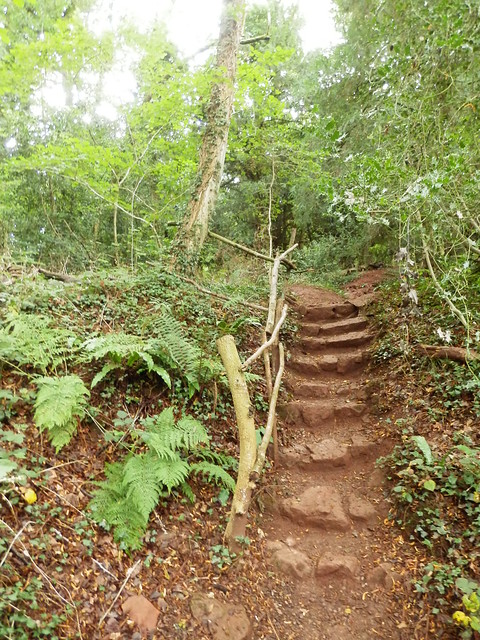The image depicts a serene woodland scene on a clear, non-rainy day with a sky partially filled with clouds. In the foreground, slightly to the right, lies a dirt path accentuated by a series of primitive stone steps, seemingly haphazardly embedded into the natural slope, creating a slightly elevated trail. These stones, matching the light brown hue of the path, guide the eye upward and are flanked by a handcrafted railing fashioned from fallen wood and branches, ingeniously blended into the natural environment.

The surrounding area is lush with various shades of green foliage, abundant with trees, sticks, weeds, and brush. The left and right sides of the path are densely populated with shrubs, vines, and underbrush, contributing to the natural, untouched feel of the woods. Scattered rocks and palm fronds lay amidst the dirt, enhancing the raw, unmanicured ambiance of the trail. In the background, the image reveals the vibrant green of the trees and the medium reddish-brown of the bare earth, with a glimpse of the bright, somewhat glary sky towards the top left. The overall scene is evocative of a typical nature walk through a forest trail, rich in natural elements and teeming with a variety of textures and colors.